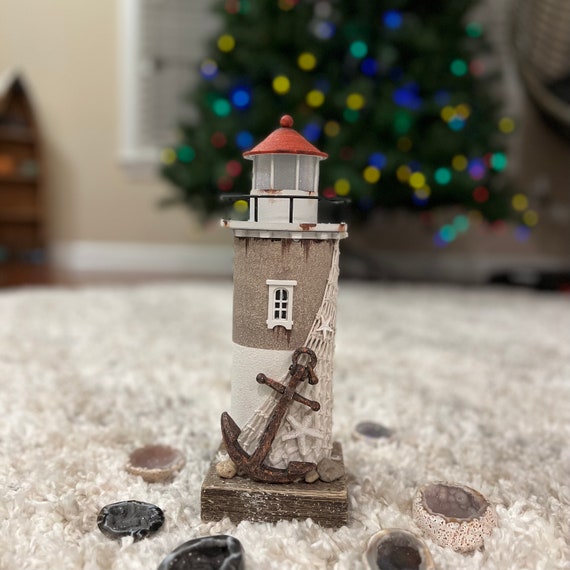The image is a full-color, vertically rectangular photograph taken indoors, clearly staged and without a distinctive background. In the top half of the frame, there's a heavily blurred Christmas tree adorned with twinkling, multi-colored lights—blue, green, and yellow. To the left of the tree is a window with white framing and drawn blinds, and in the far left, a glimpse of a bookshelf can be seen. The room has tan walls and white woodwork.

Centering the composition is a detailed, decorative lighthouse figurine positioned on a white, plush carpet. The lighthouse, seated on a taupe wooden base, features a prominent brown anchor at its base, slightly slanted, and rising about a third of the way up. Surrounding the anchor are small rocks and a rope net adorned with starfish. The lighthouse itself is primarily white at the bottom, transitioning to taupe in the middle section where a small white-framed window is visible. The roof of the lighthouse is red, and a black railing encircles the top where a light would typically be housed.

The intricate details of the lighthouse and its nautical decorations make it the focal point against the blurred yet festive backdrop of the Christmas tree, capturing an intimate and festive indoor holiday scene.